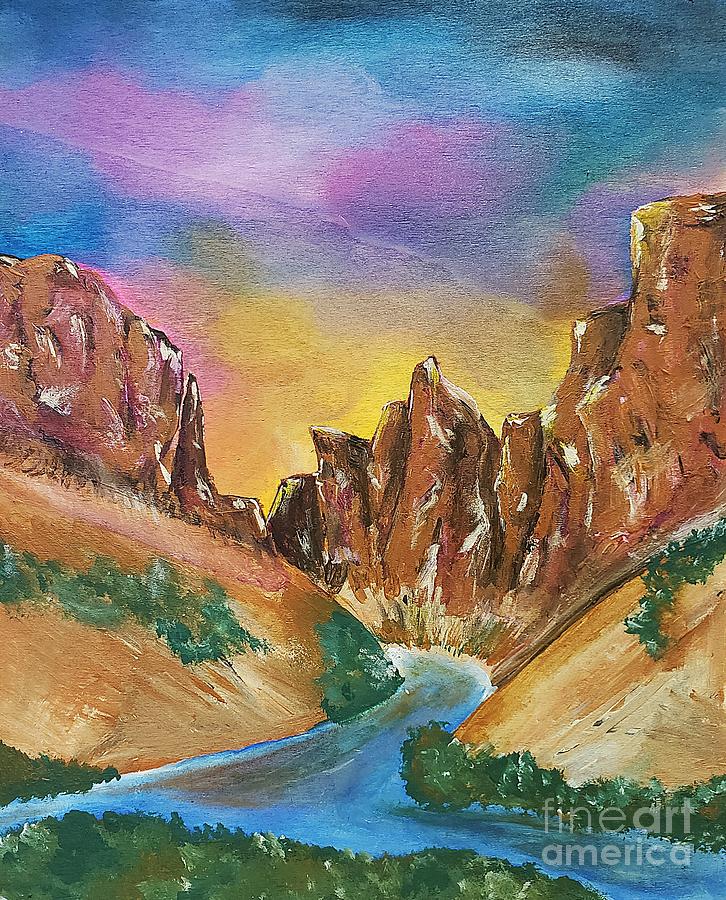This detailed painting depicts a serene desert landscape featuring a network of canyons much smaller but somewhat reminiscent of the Grand Canyon. A meandering river runs prominently through the middle of the scene, separating robustly massive brown and gold-tinged bluffs and hills, with specks of white detailing adding texture and depth. The foreground emphasizes the river's flow through verdant patches and scattered greenery over predominantly sandy, brown terrain. The sky is a vibrant tapestry, transitioning from yellow and orange near the horizon to shades of blue and purple higher up, hinting at either sunrise or sunset. A subtle hint of green is interspersed among the celestial colors, enriching the overall palette. In the bottom right corner, a partially see-through and gray watermark reads "Fine Art America," attesting to the painting's origin. This artwork, likely created with colored pencils or another medium, exudes the refined skill of a professional artist, capturing the tranquil beauty and mystique of a desert river landscape.